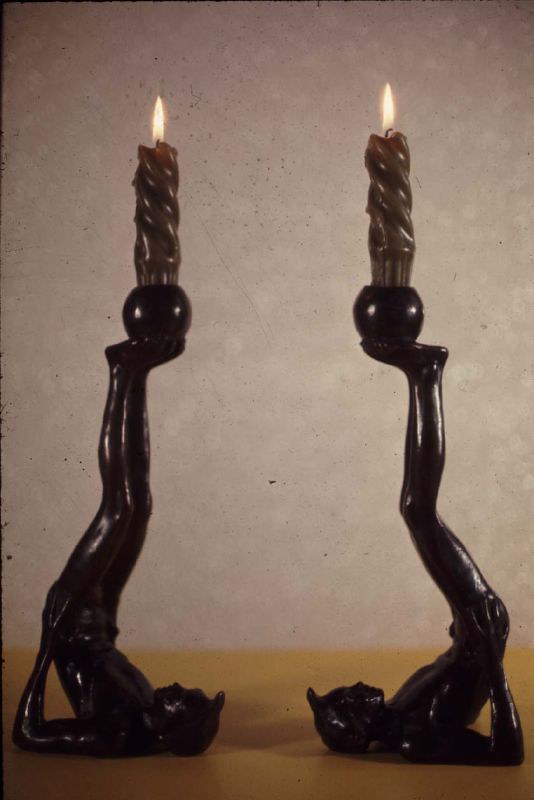In this color photograph, which has the muted hues and scratched surface typical of an old slide, two identical black candlesticks shaped like human figures are prominently displayed. The candles are nestled in round balls at the tops of the figures' feet. Each figure is posed in a yoga-like position, with their heads and shoulders resting on a light orange or beige surface, their backs arched, arms supporting their hips, and legs extended upwards. The votive candles are halfway burned and have a swirling pattern around them, with delicate flames flickering. The scene is set against a distant white or light grayish wall, highlighting the intriguing and artistic design of the candle holders. Despite the picture's age and the presence of specks that suggest it's from the mid-20th century, the composition remains clear, placing the candle holders head to head, just a few inches apart.